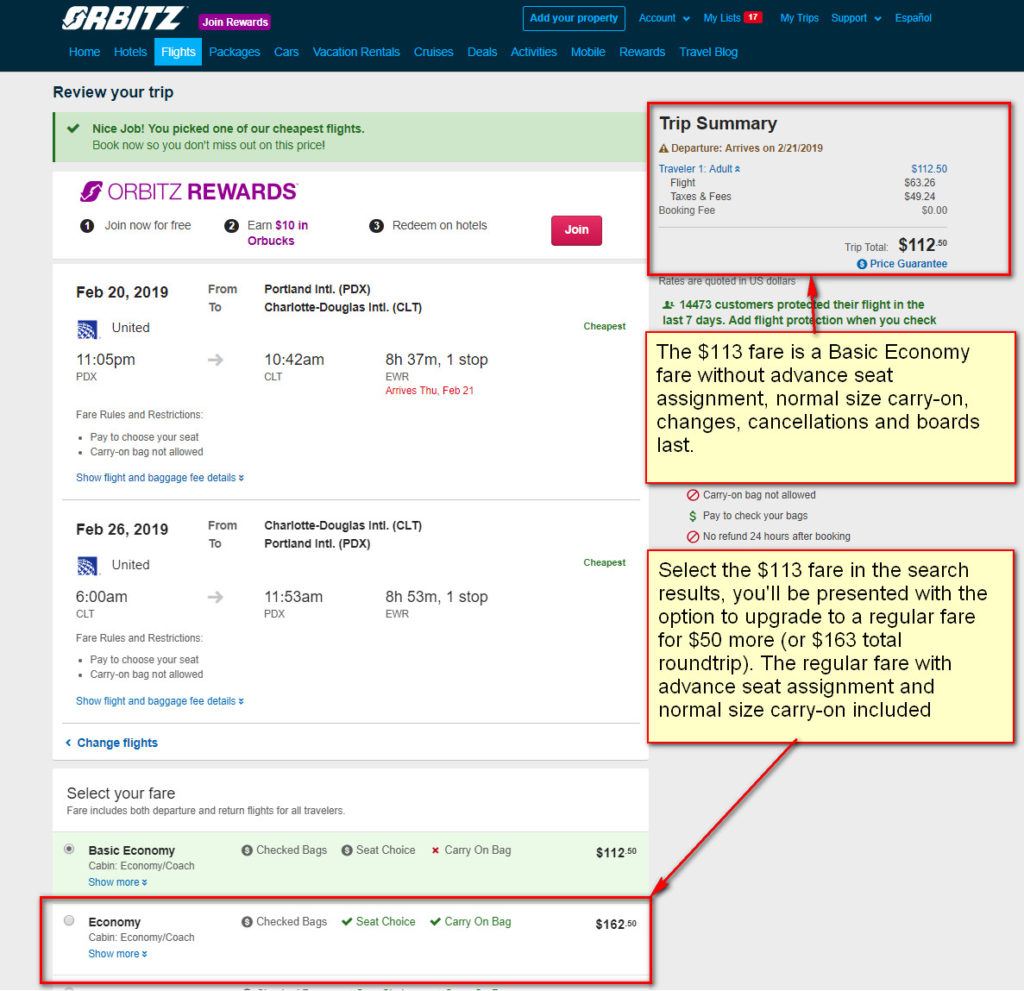"Screenshot of an Orbitz booking page, detailing various options and information for a flight reservation. The top navigation bar includes options like 'Join Rewards,' 'Add Your Property,' 'Account,' 'My List,' 'My Trips,' 'Support,' 'Espanol,' 'Home,' 'Hotels,' 'Flights,' 'Packages,' 'Cars,' 'Vacation Rentals,' 'Cruises,' 'Deals,' 'Activities,' 'Mobile,' and 'Travel Blog.' The 'Flights' section is selected.

The main content area features a summary of the user’s selected flight itinerary. The trip details display the departure and arrival information, highlighting a departure date of February 21, 2018, for one adult traveler. The fare breakdown shows the cost of the flight at $63.26, taxes and fees at $49.24, totaling $112.50. An option to protect the flight for an additional fee is noted, as well as a price guarantee claim that 1,4473 customers have protected their flights in the last 7 days.

Further down, there is information about the fare type, mentioning that it is a basic economy fare without advance seat assignments, standard-size carry-ons, and limited change or cancellation options. Users are prompted to select the $113.00 fare or upgrade to a regular fare for $50.00 more, totaling $163.00, which includes events, seat assignments, and carry-on bags. Additional options related to economy cabin, baggage, seat choices, and various taxes are also listed."